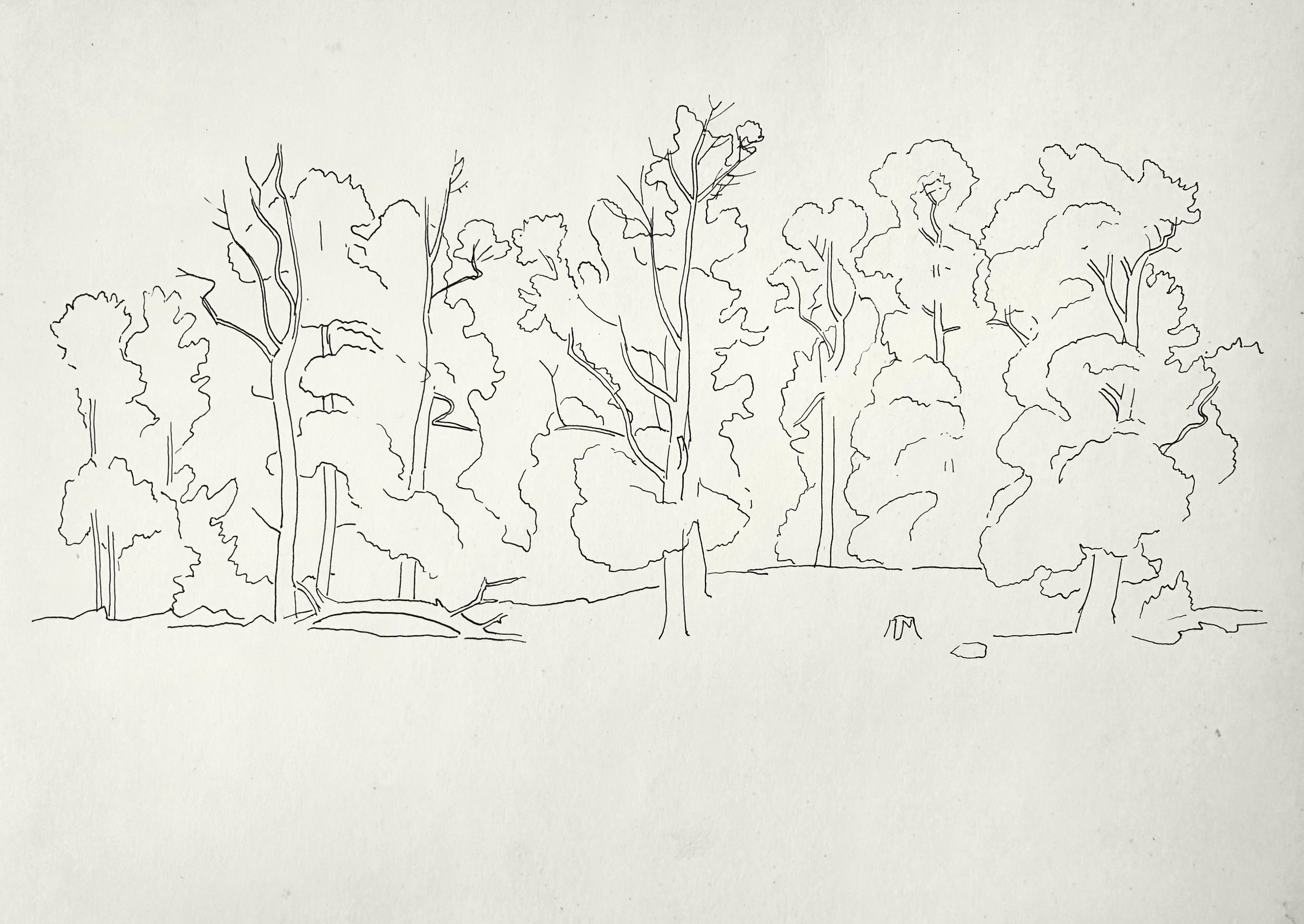This hand-sketched ink drawing depicts a sparse yet realistic tree line against an off-white background. Executed in black ink or pencil-like strokes, the sketch employs a minimalistic style with a lot of white space, leaving much to the viewer's imagination. The trees span almost the entire page, which is a horizontal rectangle close to a square in shape. Some trees are bare, while others have loosely outlined foliage, all drawn with very thin, wispy lines that suggest rather than detail. The ground is dotted with small circles representing rocks and stumps, adding subtle complexity to the otherwise empty scene. Despite the lack of color, the detailed yet understated execution captures a neutral, almost ethereal forest setting.